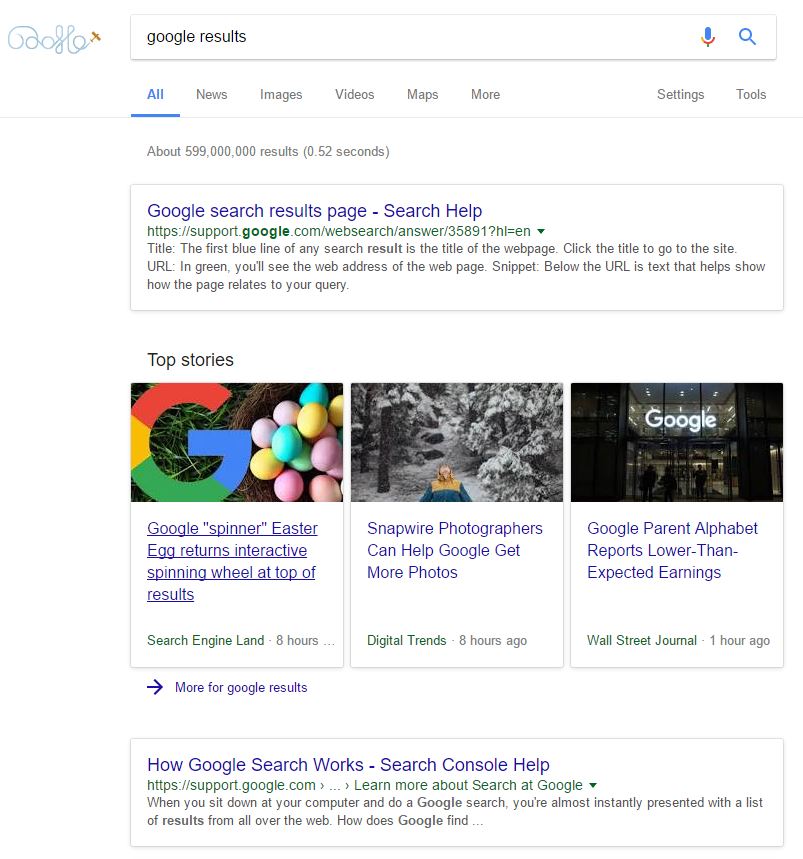The image depicts a Google search results page. At the top is the familiar Google search bar displaying "Google Results." Below the search bar are the tabs: All, News, Images, Videos, Maps, and More, alongside Settings and Tools options. The "All" tab is highlighted, indicating it is the active filter. The page shows a search result count of approximately 599 million, generated in 0.52 seconds.

The first result is titled "Google Search Results Page, Search Help" with information pulled from Google Support. Below this, a section labeled "Top Stories" showcases three news thumbnails. The first image features the Google logo and colorful eggs, captioned "Google Spinner Easter Egg Returns Interactive Spinning Wheel at Top of Results." The second image shows a woman in snowy surroundings, with text stating "Snap Wire Photographers can help Google get more photos from digital trends." The third thumbnail presents Google Headquarters, accompanied by the title "Google Parent Alphabet reports lower than expected earnings" from the Wall Street Journal.

An option to view "More from Google Results" appears beneath the Top Stories section. Further down, another search result titled "How Google Search Works, Search Console Help" provides additional support information from Google.

In the top left corner, the Google logo is stylized in a playful Doodle format, resembling an airplane leaving a trail that forms the word "Google."